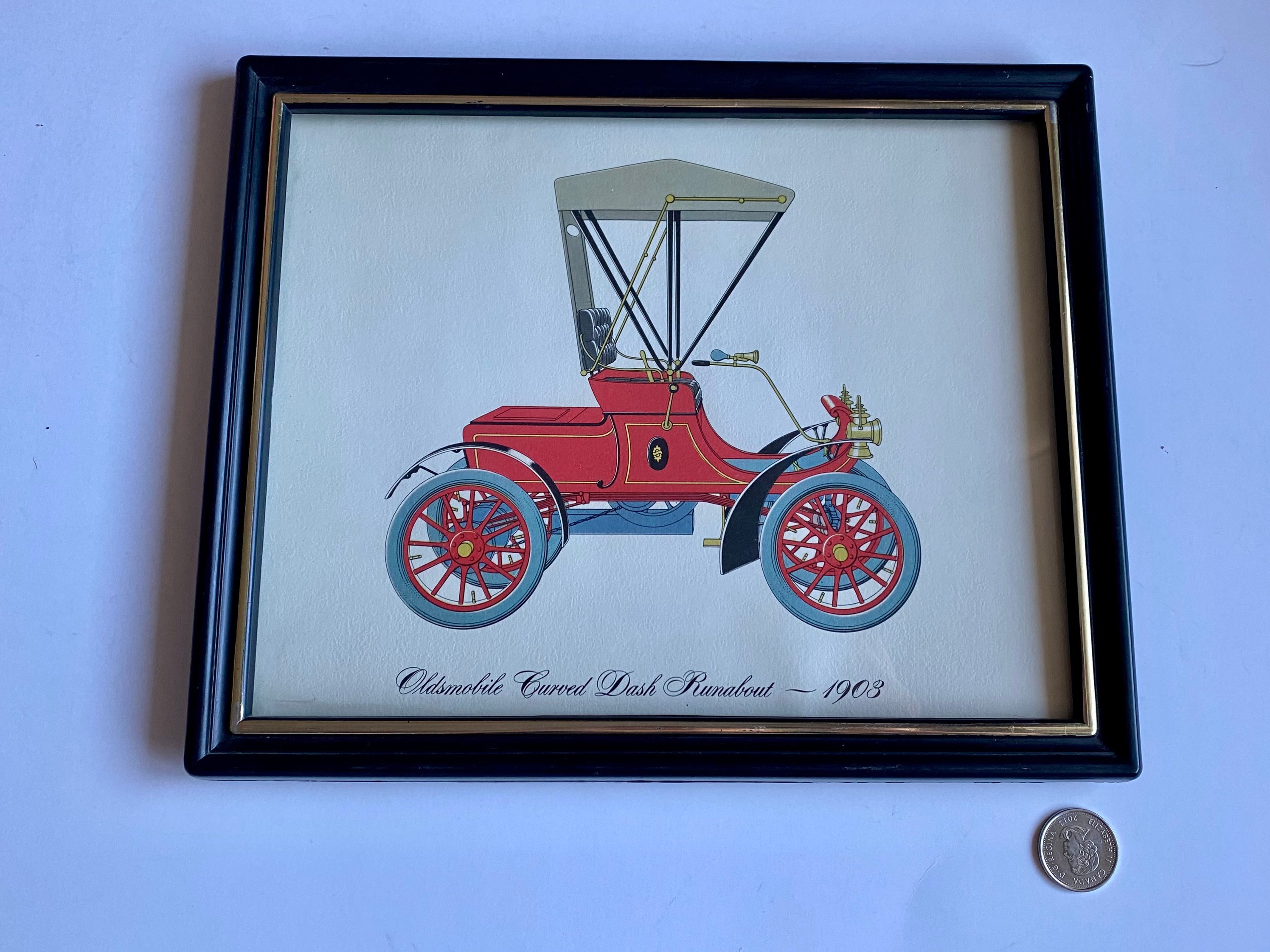The image depicts a detailed painting of an antique vehicle labeled "Oldsmobile Curved Dash Runabout 1903." The vehicle, reminiscent of an old-fashioned carriage or buggy, features a predominantly red body with blue wheels, underlined with red rims and grey tires. It boasts a black leather seat covered by a beige or khaki-colored canvas top, and is adorned with gold accents, especially on the headlights and metal trim. A small blue horn is mounted on it. The artwork is framed in a black frame with gold detailing, set against a white background or tabletop. A silver coin, identified as a 2013 dime with President Roosevelt's profile, is placed at the bottom right corner of the frame, presumably to represent the artwork's scale.